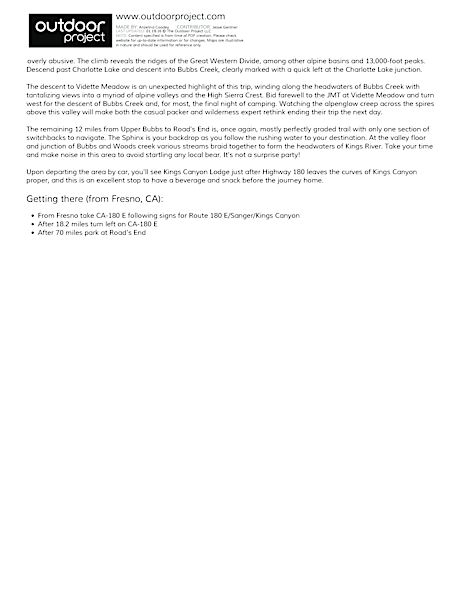This image showcases the homepage of Outdoor Project's website, www.outdoorproject.com. At the top of the page, the company's URL is displayed prominently. While the company provides a detailed description of their mission and activities, the text is printed in very small font, making it difficult to read. The content highlights Outdoor Project's focus on the Great Western Divide, detailing its geographical and historical significance. It also offers specific directions from Fresno, California, advising travelers to turn left onto Highway 180 East for the remaining 12 miles. The site suggests that visitors can meet with the company in person, indicating they have a physical shop. However, it lacks an interactive map feature, such as a link for users to input their addresses or a visual map with pins marking significant locations and surrounding areas. Adding such an element would enhance the user experience by simplifying navigation and trip planning.